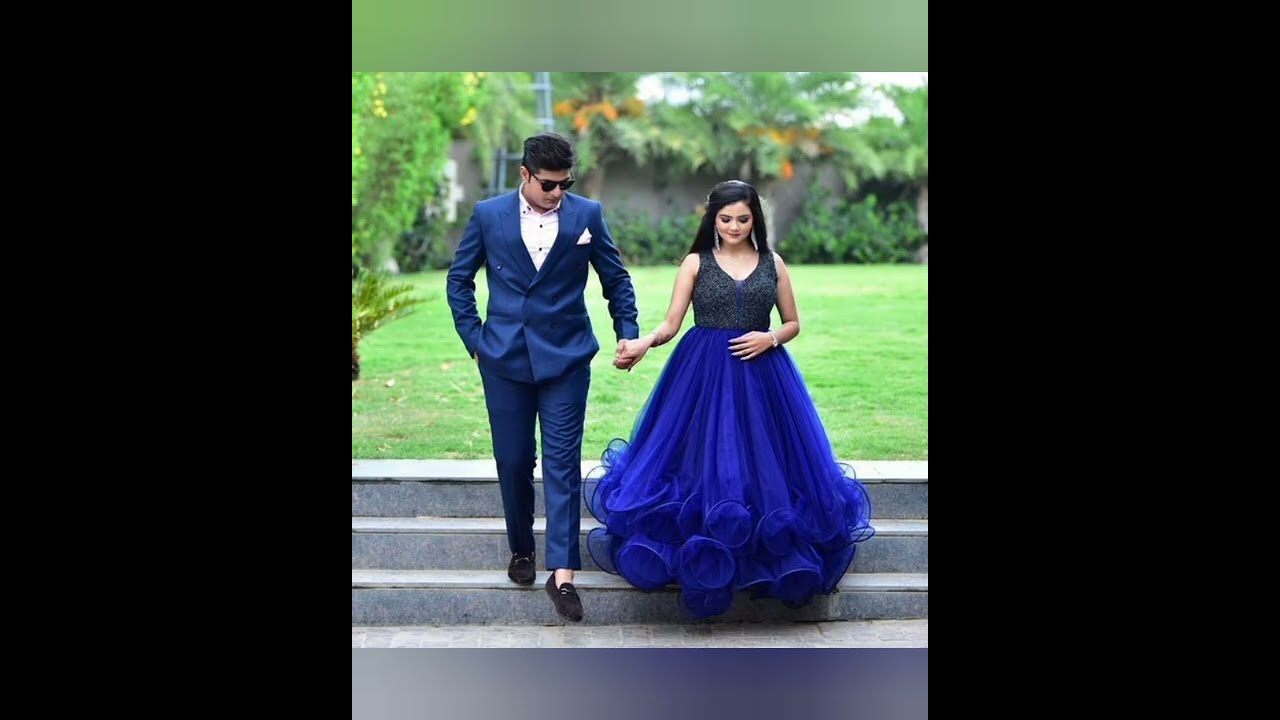In this image, a young couple, appearing to be in their twenties, is captured walking down a stone staircase, hand in hand, hinting at a formal event such as a wedding or an elegant party. They are the focal point of the image, placed directly in the center. The man is dressed in a dark blue suit with matching pants, a white collared shirt, and black loafers without socks. He accessorizes with black sunglasses and a white kerchief neatly tucked into his pocket. His hair is short and black. The woman beside him has long, dark hair cascading down her back and is adorned with long, dangly earrings. She wears a sleeveless dress featuring a dark navy-blue, patterned top with a v-neck, and a voluminous, bright royal-blue skirt that billows as she walks, ending in delicate, spring-like coils. Both appear well-groomed, with the woman’s face visibly made up. 

In the blurred background, an outdoor setting is depicted, showcasing a courtyard with lush green grass, various plants, and a vine-covered concrete wall. This backdrop, together with the vivid colors of the couple’s attire, gives the image a vibrant and sophisticated feel. The image is bordered by solid black strips on the left and right sides, and the top and bottom have faded green and blue borders, respectively. The scene appears to be illuminated by daylight, suggesting it was taken in the middle of the day.